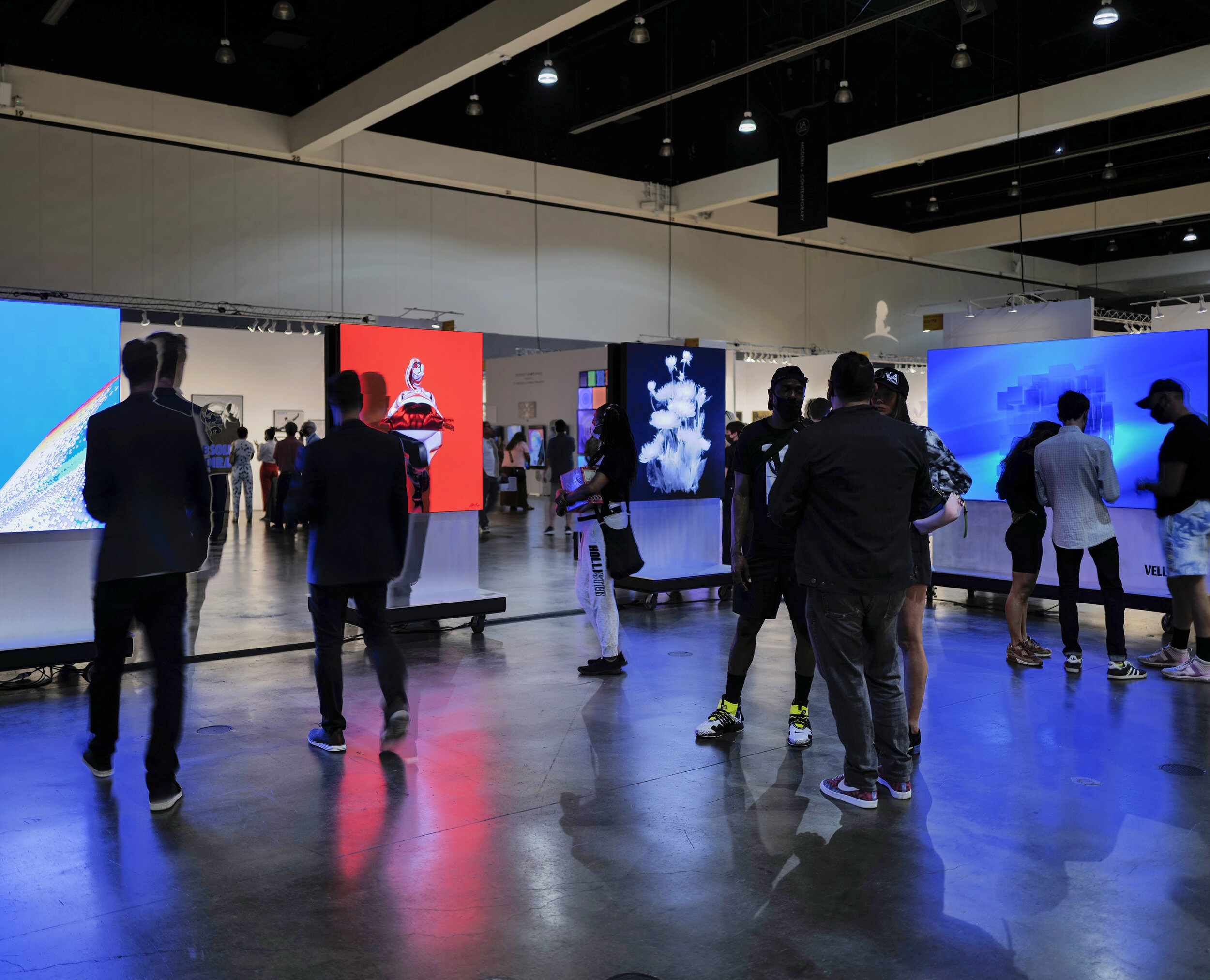The detailed image shows an exhibition likely set in a convention center or art gallery with a spacious, open layout. The environment is dimly lit, contributing to the dark ambiance with black walls and ceiling incorporating metal girders and spotlights. The flooring is distinctly black tile, polished to a high sheen that reflects the light emitted by digital displays around the room.

Numerous attendees, predominantly dressed in black jackets and shirts, are present, with many having their backs facing the viewer as they intently observe the displays. The crowd can be seen all around, with clusters of people gathered at various segments of the exhibition space.

There are multiple digital screens and monitors showcasing various artworks, positioned both on the walls and on rolling stands. On the left side of the image, there are three notable displays: one with a blue background and white details, another with a dark blue backdrop featuring white flowers, and a third with a vivid red background possibly depicting a person. The right side of the room features a larger screen which appears to be a significant focus, perhaps displaying a presentation relevant to the artworks, and surrounded by a small group of viewers.

In the backdrop, more screens continue to line the walls, indicating the expansive nature of the exhibition. This large area, framed by its black and grayish-white structural elements, creates an immersive setting for showcasing high-quality, detailed digital artworks that emit light, contributing further to the reflective quality of the floor. This scene encapsulates an event bustling with activity, keen interest, and a modern artistic vibe.